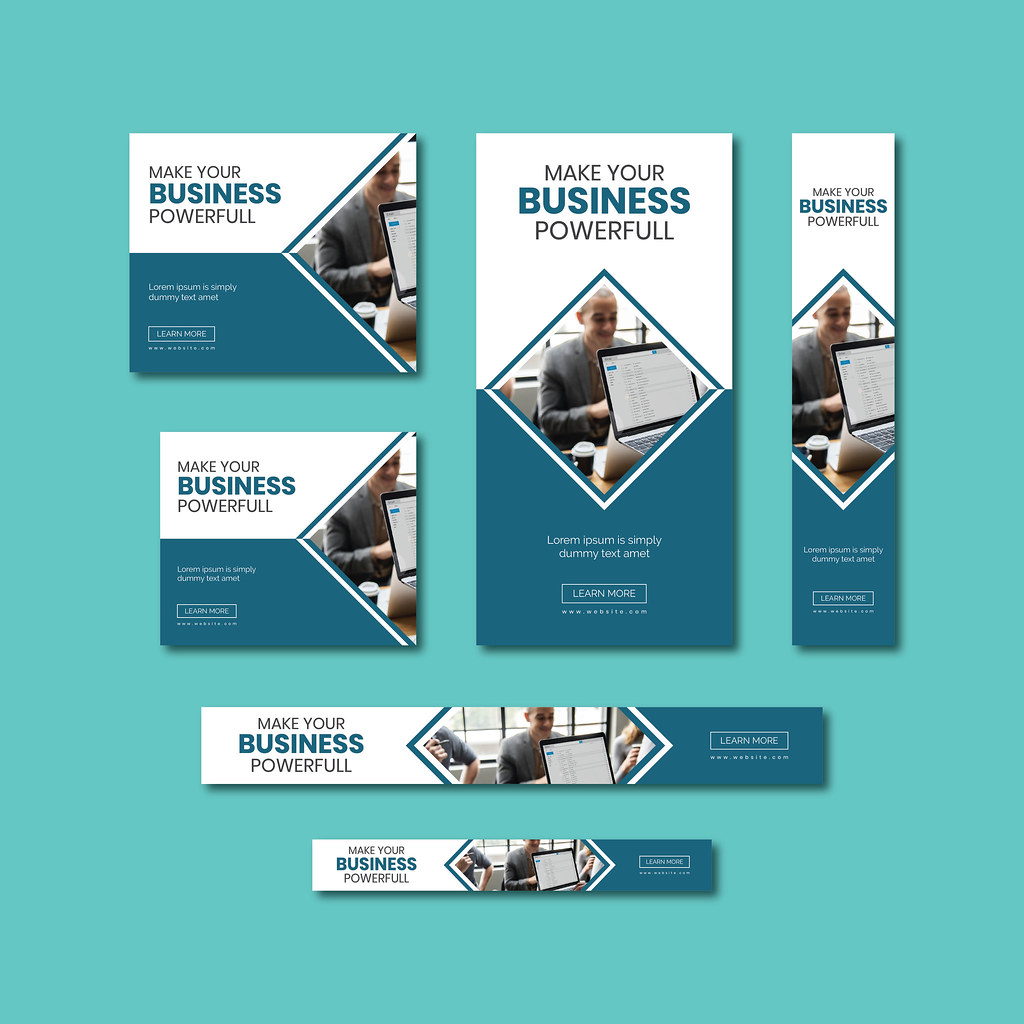The image features a teal background, showcasing six variations of the same design, each in different sizes. Each variation includes a partially white and dark teal background. On the white portion, the text reads "Make Your Business Powerful." Below the text, there is a photo of a man sitting at a table with a laptop and a cup of coffee. The man is partially obscured by the open laptop in front of him, with the screen visible to the viewer. The bottom section of the image, rendered in dark teal, contains white text displaying a standard placeholder "Lorem ipsum" paragraph. Beneath this text, there is a "Learn More" prompt followed by a website URL.